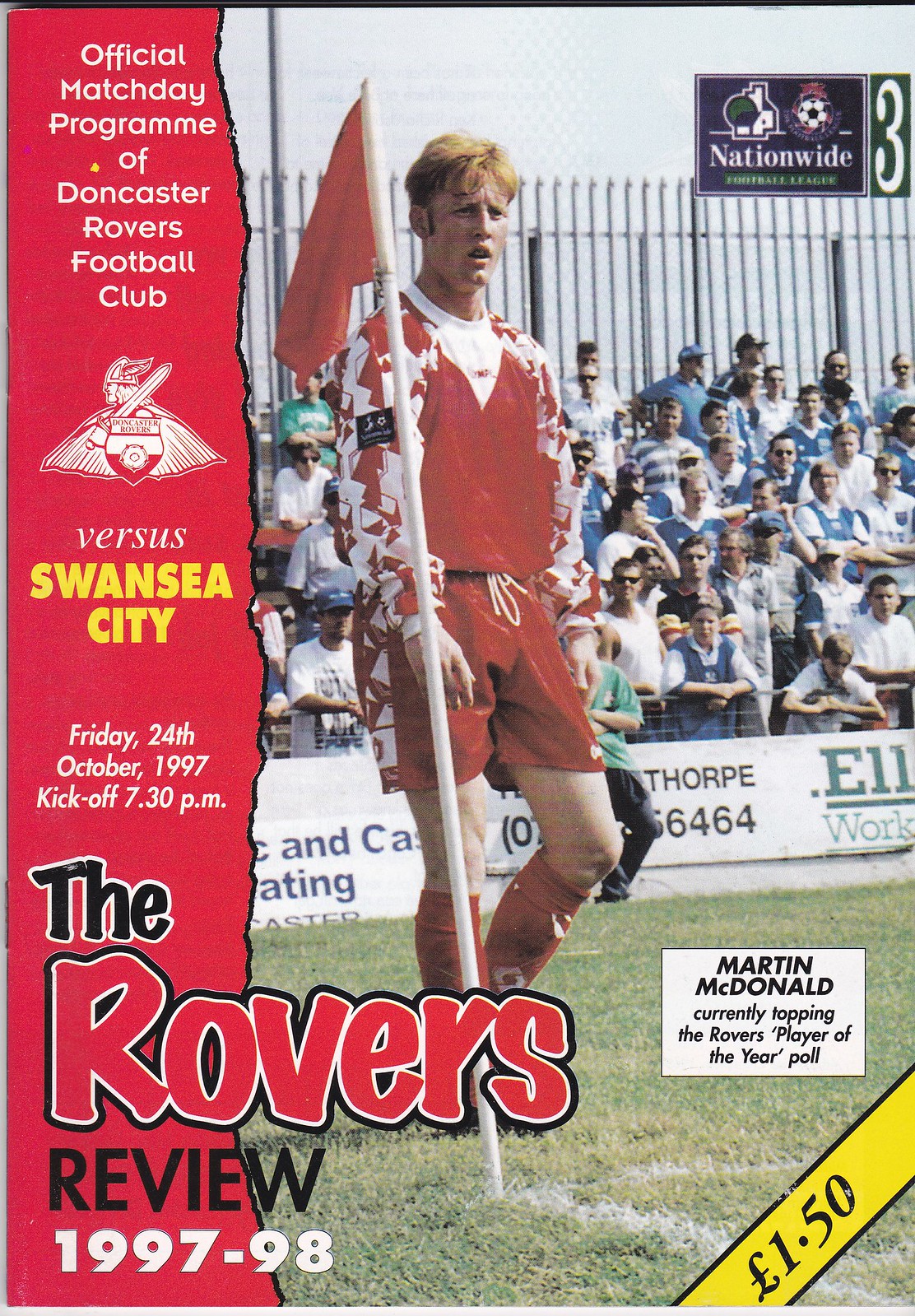This is the cover of a match day program for the Doncaster Rovers Football Club in England. The left side features a red vertical band with white text that reads, "Official Match Day Program of Doncaster Rovers Football Club." The iconic Doncaster Rovers logo, portraying a Viking character in red and white, is displayed prominently. Beneath the logo, it states in yellow text, "Versus Swansea City," indicating their opponent for the game. The date, "Friday 24th October 1997," and the kickoff time, "7.30 p.m.," are written in white text below this. Toward the bottom, it says in large letters, "The Rovers Review 1997 to 98," with the word "Review" in black.

The right side of the cover shows a vibrant photograph of a player in a red uniform, standing near an out-of-bounds flag. Behind him is a crowd of spectators, visible through a metal fence. On the lower right, within a yellow band, the price of the program is stated as "1.50 pounds." Additionally, it mentions "Martin McDonald," the player currently leading in the Rovers' Player of the Year poll.